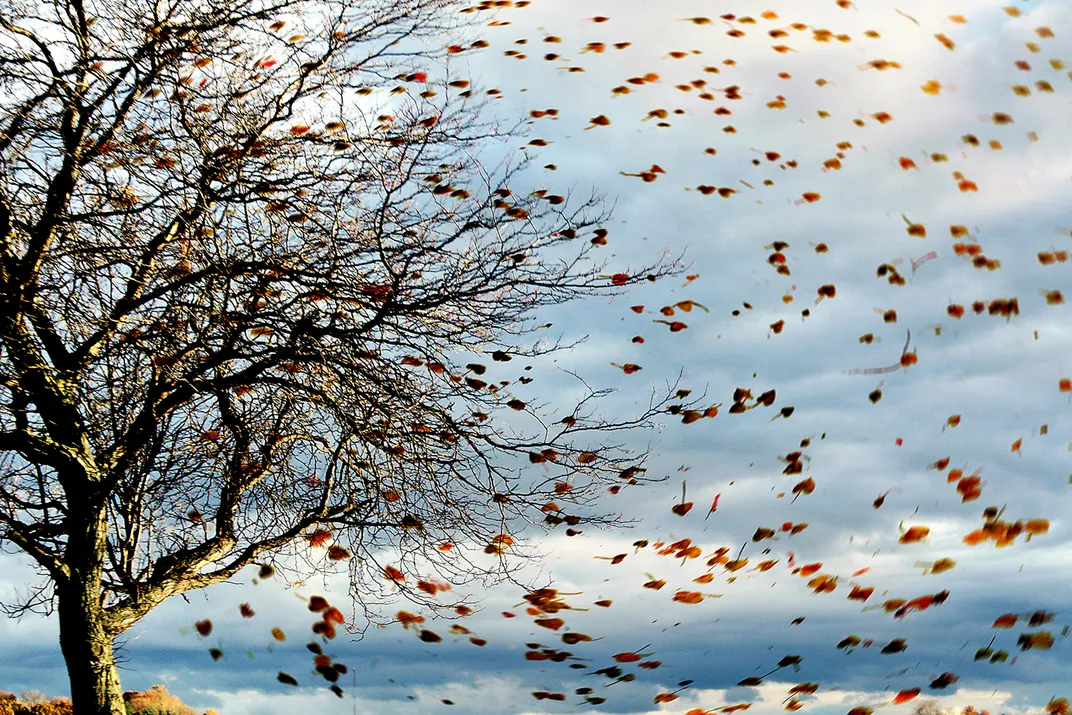The image captures an almost surreal outdoor scene dominated by a photorealistic, large, leafless tree with tangled and winding branches on the left side, taking up about a third of the frame. The backdrop is primarily a blue sky densely packed with dark, reflective clouds, leaving little clear sky visible. The central focus of the photograph is the dynamic movement of reddish-brown leaves caught in a powerful wind, creating a spiral or circular motion across the right side of the image. This motion gives the leaves a blurred, warped appearance, emphasizing their rapid flight. The scene also includes a small patch of dark dirt or rock under the tree, though it is not a significant part of the composition. The image contains neither writing nor any people, animals, buildings, or mechanical objects, making the natural elements the sole subjects of this vivid, expressive photograph.